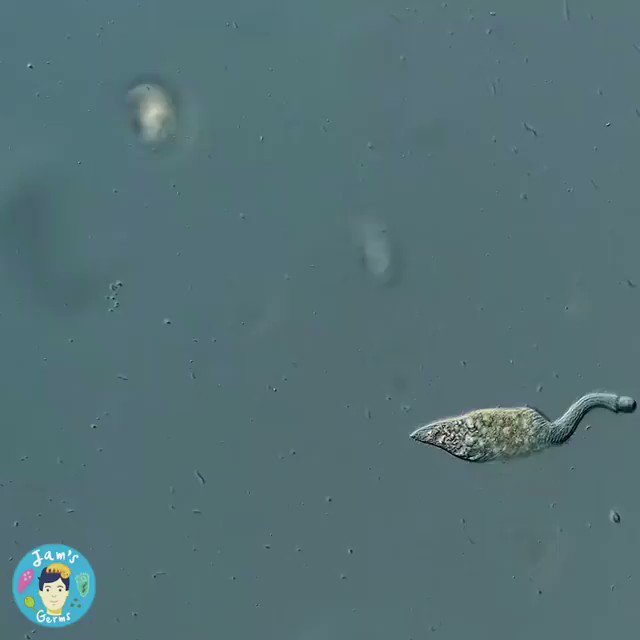The image is an up-close photograph that appears to be taken under a microscopic lens, depicting a microorganism floating in a bluish-gray liquid. The microorganism has a distinct arrow-shaped head packed densely with various internal structures, possibly organelles, and is situated in the lower right area of the image. It features a long, upward-curving tail that ends in a small ball-like structure. The background is speckled with numerous black and white particles.

In the lower left corner, there is a blue circle with a cartoonish head of a man with short black hair at its center. Above the head, the word "JAMS" is written in white, and below, it reads "GERMS." This circle also contains a pink oval-shaped germ, a green round germ, and a green triangle-shaped germ. The image overall has a scientific feel to it, with the central focus being the clear, bluish-gray microorganism, resembling a microscopic organism such as a germ or amoeba, amidst a backdrop that conveys a watery environment.